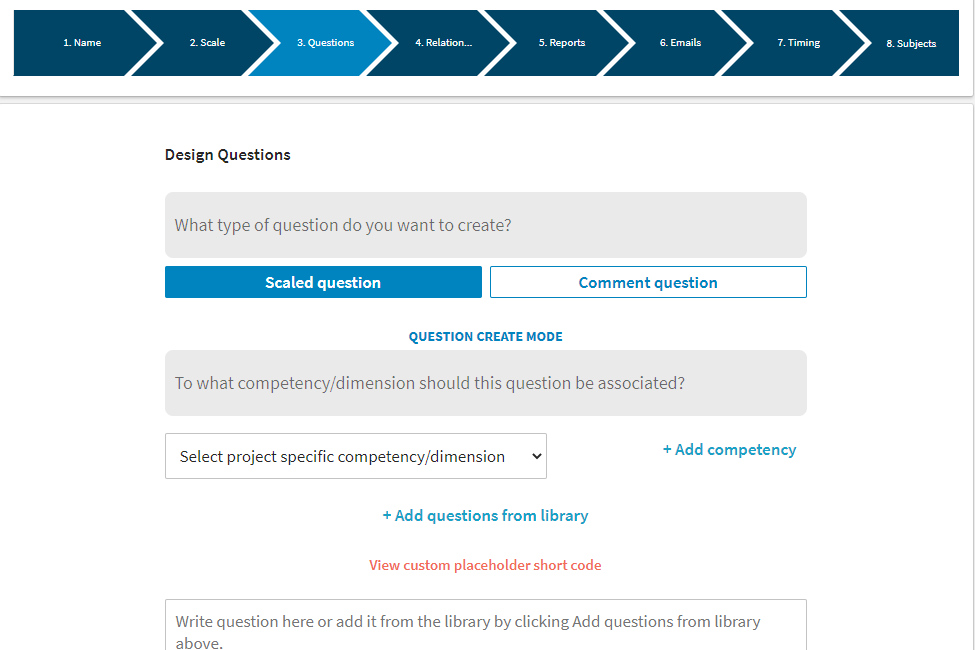The webpage displays an eight-step workflow, each step labeled and color-coded. The navigation bar, featuring navy blue tabs with white fonts, lists the steps sequentially: Name, Scale, Questions, Relation, Reports, Emails, Timing, and Subjects. The current active step, highlighted in light blue, is "Questions."

Below the navigation bar, against a white background, is a section titled "Design Questions." Here, users are prompted with the query, "What type of question do you want to create?" Two buttons are presented as options: a light blue button with white text labeled "Scaled Question" and a white button with blue text labeled "Comment Question."

Further down, blue text reads "Question Create Mode," accompanied by a grey tile prompting, "To what competency/dimension should this question be associated?" A dropdown menu below this tile is currently set to "Select project-specific, competency/dimension." Users have the option to add new competencies through a plus link adjacent to the dropdown.

Additionally, there is a plus link allowing users to add questions from a pre-existing library. Directly below this, in blue font, is a link that says "View custom placeholder shortcode."

At the bottom of the page, within a bordered box, is a message prompting users to "Write question here or add it from the library by clicking 'Add questions from library' above."